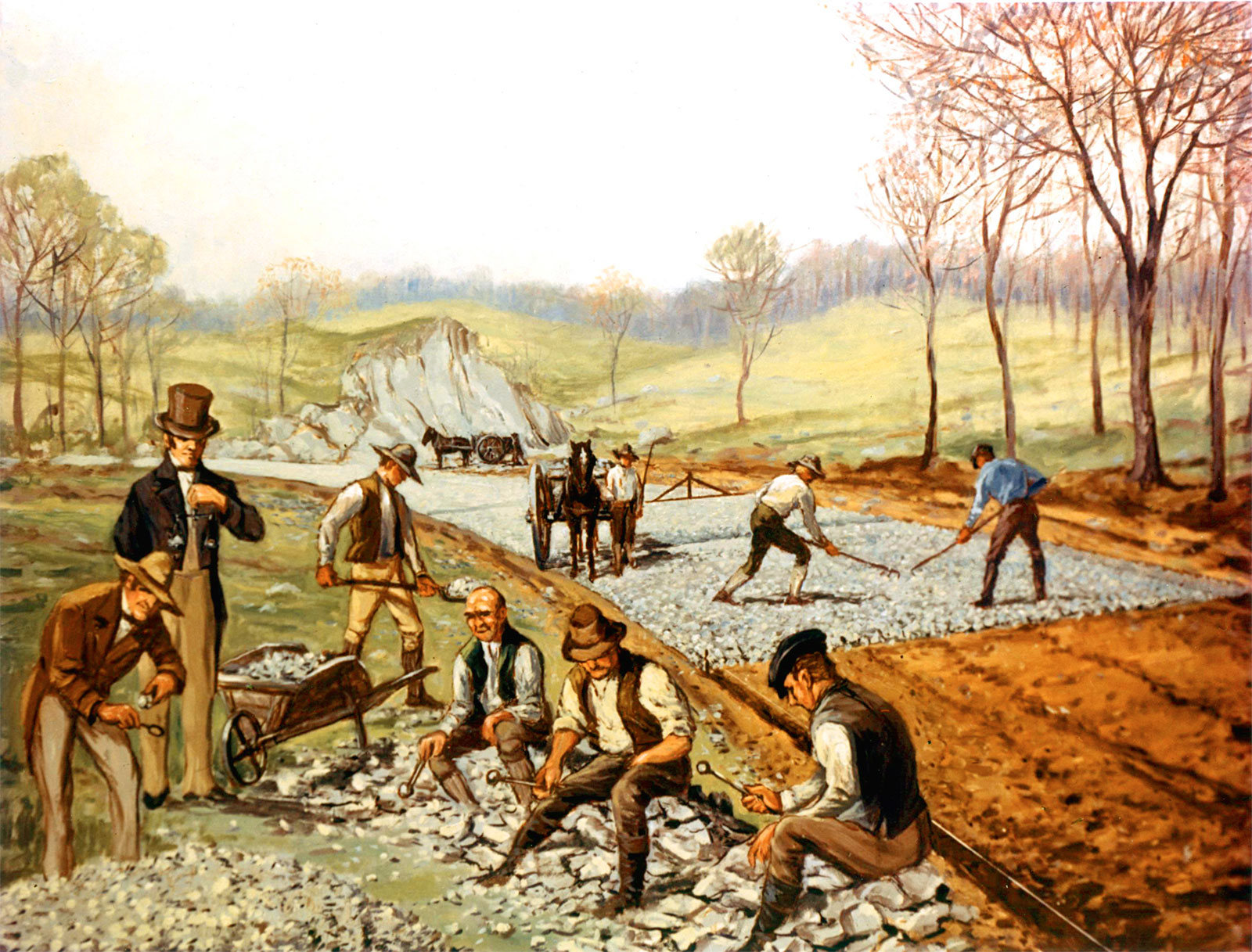This painting, a horizontal rectangle with a historical tone, depicts an industrious scene of about 10 men engaged in hard labor on a railroad track construction, set amidst a picturesque landscape with fields and a backdrop of dense trees. The men, dressed in predominantly dark and earthy tones characteristic of the 1800s—including brown vests, shirts, pants, and some navy elements—are captured in various states of activity. Some are actively working with shovels and wheelbarrows filled with stones, while others take a respite, seated on rocks or examining them. The scene is further detailed with a couple of horse-drawn carriages and a man in a tall top hat standing beside one. The artwork, in muted, quieter tones of green, brown, and gray, also features dark-colored horses and subtle greenery in the background, enhancing its serene yet hardworking atmosphere.